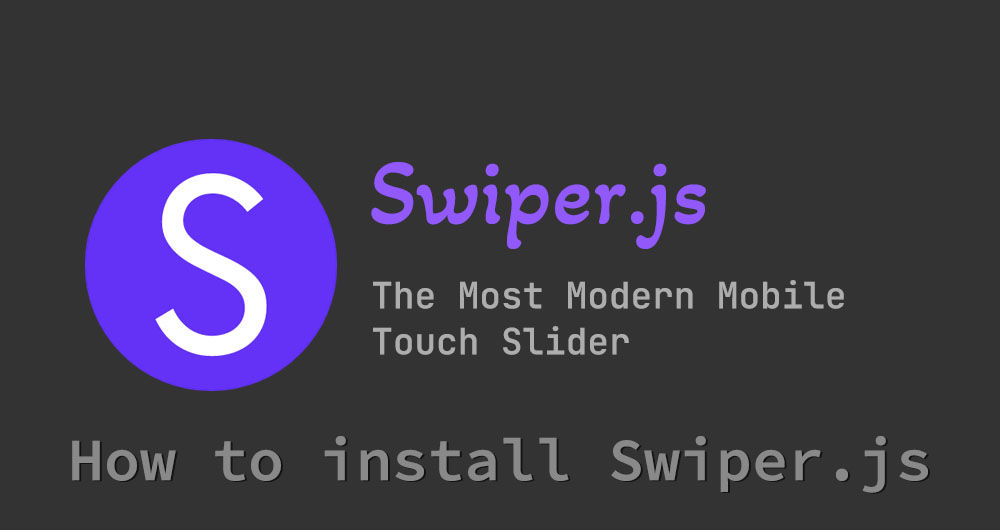This is a detailed descriptive caption for the given image:

---

The image is a screenshot of a promotional banner ad. The ad features a black rectangular background with a prominent blue circle in the center, containing a white letter "S". Next to the circle, in bold purple letters, is the text "swiper.js". Below it, in smaller gray letters, is the tagline "The most modern mobile touch slider." Further down, also in gray letters, is the phrase "How to install swiper.js." The ad focuses on promoting swiper.js, likely a JavaScript library for creating touch sliders on mobile devices.

---